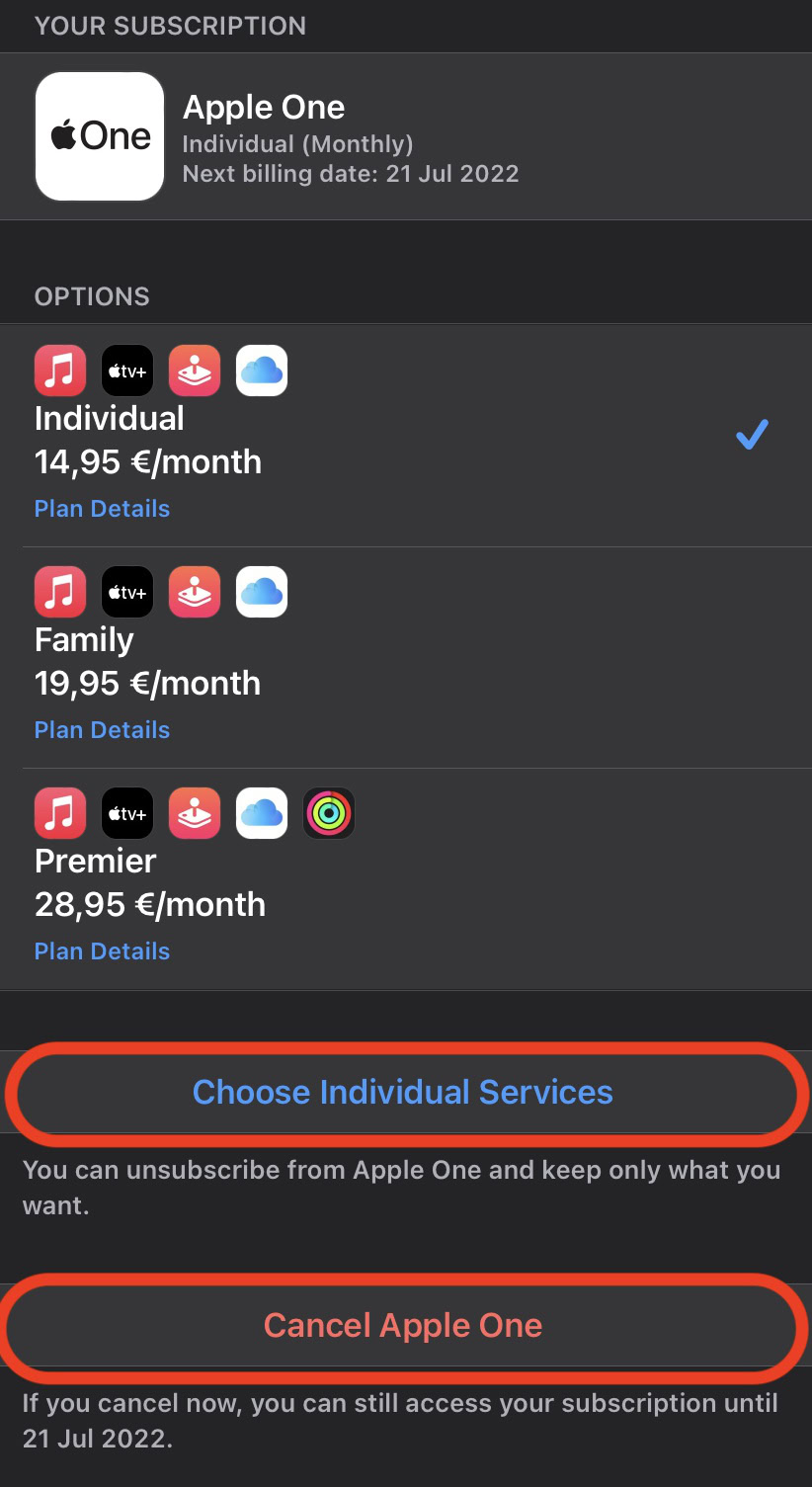The image is a dark mode screenshot of a mobile landing page detailing subscription information for Apple One. At the top, it prominently displays the heading "Your Subscription," followed by the Apple One logo thumbnail. Beneath this, it lists the subscription details: "Individual Monthly" with the next billing date specified as July 21, 2022.

The entire interface utilizes a dark theme with black or very dark gray backgrounds, contrasting with colorful thumbnails or icons for various sections. Below the subscription details, there's a section labeled "Options" featuring four icons likely representing services such as Apple Music, iCloud, and Apple TV+.

Following this, the pricing plans are outlined:
1. **Individual Plan** priced at 14.95 euros per month, with a blue check mark indicating it is currently selected. Next to this, there's a clickable option for "Plan Details."
2. **Family Plan** priced at 19.95 euros per month, similarly accompanied by the same service icons and a clickable "Plan Details" option.
3. **Premier Plan** priced at 28.95 euros per month, featuring the same service icons along with an additional icon consisting of concentric circles in red, yellow, green, and black. This option also includes a clickable "Plan Details" button.

Below the pricing plans, there's a highlighted prompt, "Choose Individual Services," encased in a red oval, indicating users can opt to customize their subscription. There's also an option to "Unsubscribe from Apple One and keep only what you want," emphasizing the flexibility of the subscription management.

At the very bottom, a red-outlined oval button labeled "Cancel Apple One" is present, with a note informing users that if they cancel immediately, they will retain access to their subscription until July 21, 2022.